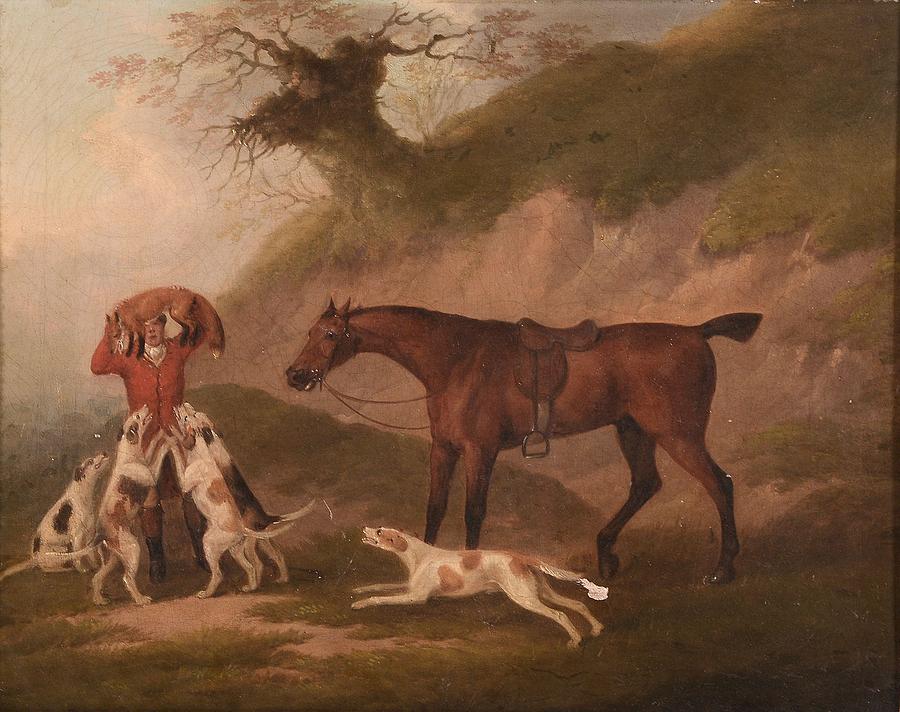This detailed traditional 19th-century oil (or possibly acrylic) painting depicts an English hunting scene. At the center stands a hunter in a red long-sleeved blazer, horse-riding jacket, shorts, and boots. He holds a red fox above his head, and its condition—whether snarling or dead—is ambiguous. Surrounding the man are five hunting hounds, white with brown and tan spots: three are standing with their paws on his waist, one is sitting at his feet, and another is running towards him. To his left is a brown horse, equipped with a saddle and bridle, facing left in profile with its neck extended and teeth visible. Its tail appears notably short.

In the backdrop, a hillside emerges, covered in patchy green moss and grass. Rising from the hill is a tree with an unusual structure, where it appears bushy at the base but tapers off with sparse branches, almost looking like it’s growing upside-down, with roots seemingly sprouting from the top. The sky above is a pale blue, contributing to the scene’s serene yet lively atmosphere. The painting itself shows signs of age with visible cracks. The ground beneath the figures is a mix of green and brown patchy grass, emphasizing the scene's dynamic and somewhat rustic setting.